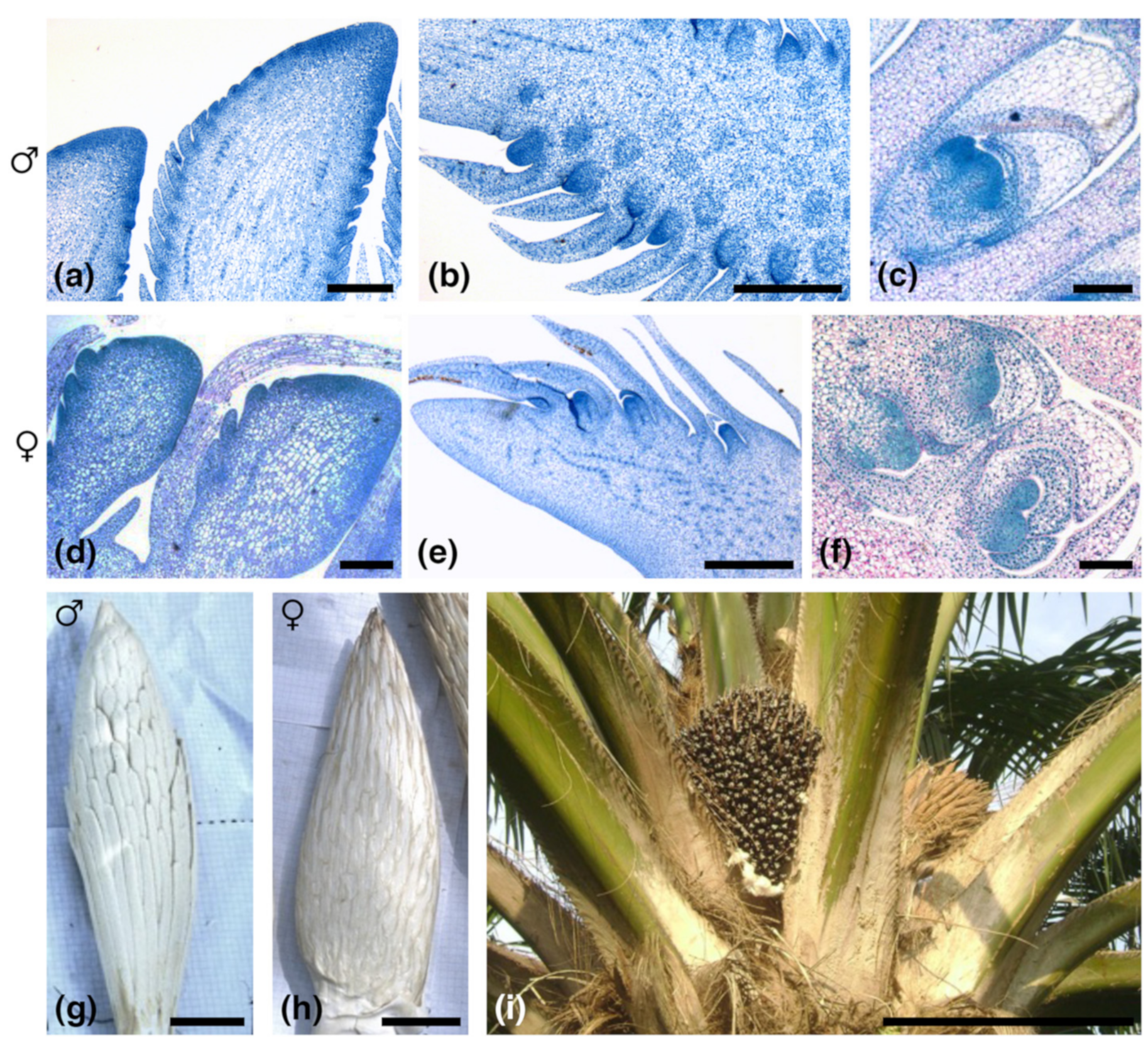The image showcases nine distinct sections labeled from A to I, divided into three rows of three images each. The top two rows feature microscopic views of various parts of a palm tree, depicted in an array of colors including blue, pink, white, green, tan, and brown. Labels next to each image identify them with either a male or female symbol. Images A, B, and C show detailed microscopic structures, with A resembling blue feather-like shapes, B displaying a creature with multiple legs, and C looking like an eyeball. Images D, E, and F continue to present microscopic views of palm parts. The bottom row shifts to regular images of the palm tree components, with G and H highlighting palm leaves or buds, and I showing a comprehensive view of the palm tree's top. The arrangement and labeling offer a comparative study between the normal views and the microscopic examinations of the plant parts.